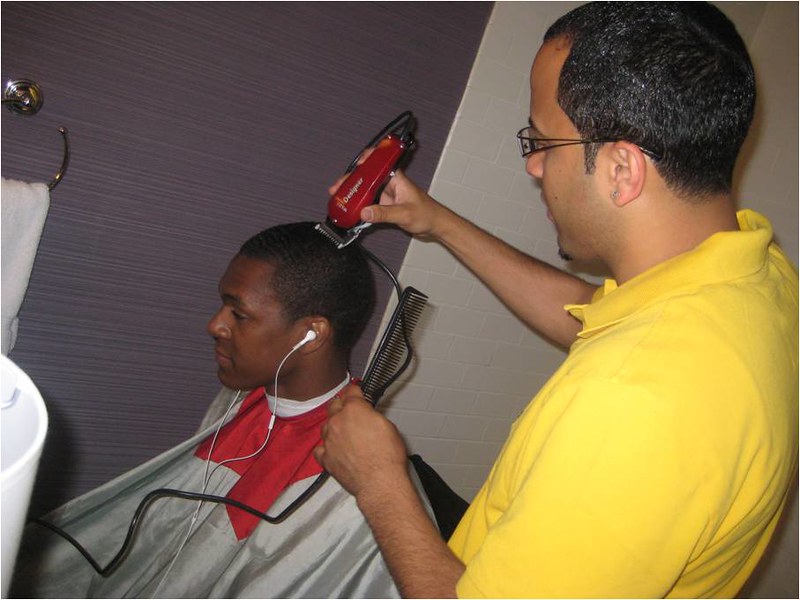In a cozy barber setup, a man with dark, short hair and glasses is seen wearing a bright yellow polo shirt as he meticulously uses a red-handled electric clipper with a silver blade to shave the head of another man. The barber's left hand holds a comb as he works. The client, an African-American man with curly, closely-cropped hair, sits in a chair with a haircut cape draped around his shoulders. He is calmly listening to music through white earphones, likely connected to an Apple device. The background features a light violet wall adorned with a striped wallpaper pattern, and a white towel hanging from a hook, adding a homely touch to the setting. In front of the seated man, there is a white sink, enhancing the authenticity of this intimate and personalized grooming scene.